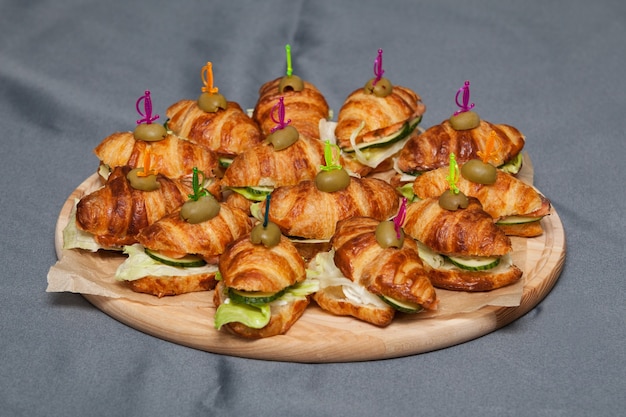This image depicts a detailed and appetizing scene of small croissant sandwiches elegantly arranged on a round wooden platter. The wooden platter, which showcases a natural light brown color with visible grain, is lined with a sheet of torn-edged parchment paper. Positioned in a landscape format, the platter rests on a gray, slightly wrinkled tablecloth that adds a casual yet refined backdrop to the setup. Each golden-brown croissant, sliced horizontally, is filled with fresh lettuce and cucumber slices, occasionally complemented by mayonnaise or even avocado. The sandwiches are uniformly topped with a halved green olive, secured in place by colorful plastic sword toothpicks, available in festive neon shades of orange, pink, yellow, and green. These swords not only hold the sandwiches together but also add a playful touch to the overall presentation.